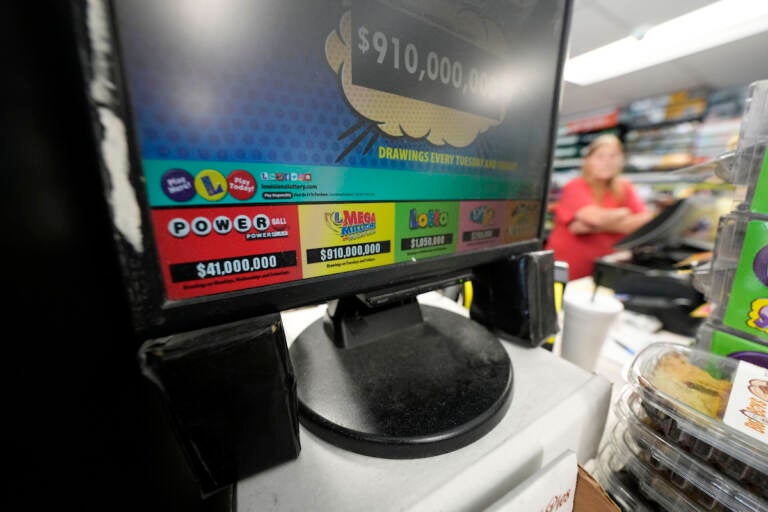This photograph, taken from the perspective of someone looking into a convenience store, captures the scene behind the counter where the cashier stands. The main focus is on a black lottery monitor, which prominently displays an impressive jackpot of 910 million dollars, alongside a note that draws take place every Tuesday and Saturday. The screen features a colorful array of lottery choices at the bottom, displaying different games in red, yellow, green, pink, and orange. There is also an aqua band on the monitor with additional lottery logos.

The background is slightly blurred but reveals a blonde-haired woman in a red shirt, leaning against a black cash register. Her arms are crossed as she attends to the counter area. Additional details such as a dusty base of the monitor and some boxed or plastic-wrapped food items stacked to the right add to the realism and everyday atmosphere of the scene, likely reminiscent of a 7-Eleven or similar convenience store.